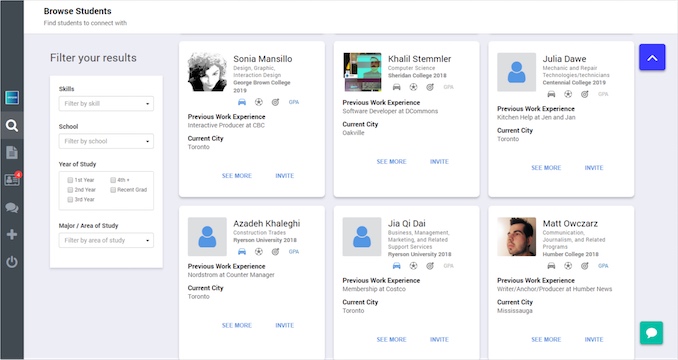The image depicts a social media website interface designed for connecting students. On the left side, there's a grey bar menu with a blue square icon and an unreadable text logo above it. Below this, there are icons: a selected search magnifying glass, an ID-like document with a red circle containing the number 4, chat bubbles, a plus sign, and a power sign.

At the top center of the layout, the text reads "Browse Students - Find students to connect with." Below this, to the left, a panel with a pink (or perhaps grey) background offers filtering options: by skill, school, year of study (with dropdowns for first through fourth years or recent graduates), and major area of study.

The main content area displays six student profile panels arranged in two rows of three. Each panel features detailed information about a student. For example, one panel showcases Sonia Mancillo, a graphic and interaction design student from George Brown College, class of 2019. This panel includes icons like a car and a soccer ball, her GPA, an "up" button, her previous work experience (Interactive Producer at CBC), and her current city (Toronto). A "See more" and "Invite" button completes the panel. The other panels follow a similar layout, providing profiles of other students with their respective details.